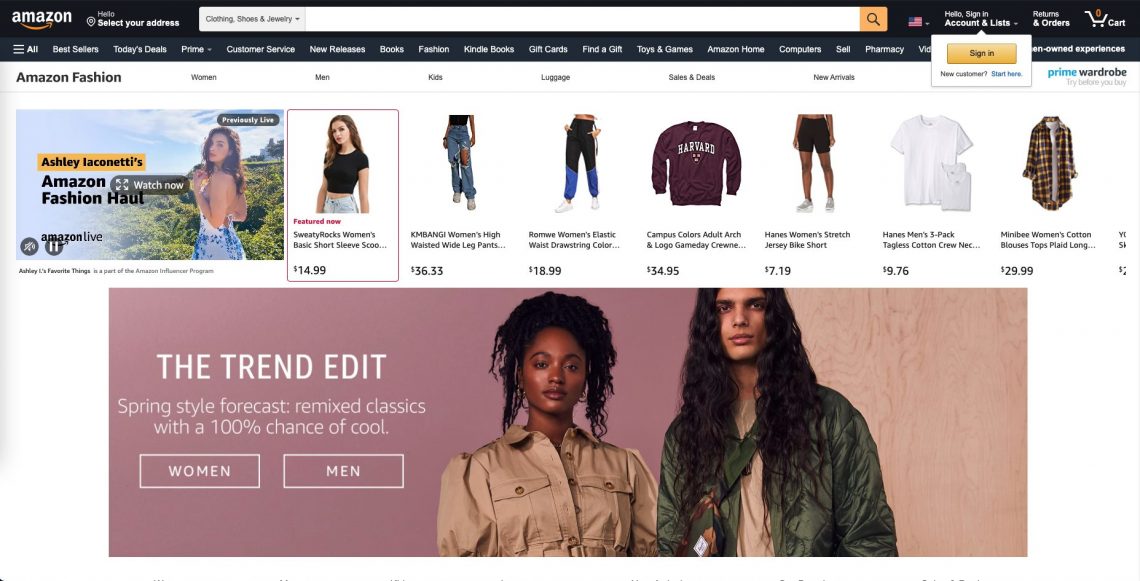This image showcases a web page from the Amazon website. In the upper left corner, the iconic Amazon logo is prominently displayed, followed by a navigation bar at the top of the page. The user has selected the "Amazon Fashion" section, which is evident from the collection of images featuring various clothing items. The page is adorned with pictures of models showcasing different outfits, with a focus particularly on pants and other apparel. The bottom half of the image features a large pink mauve-colored box labeled "The Trend Edit." In this section, there is a picture of a man and a woman. The man has notably long, black, wavy, and curly hair that is even longer than the woman's hair. He is dressed in a jacket of a deep forest green hue and has a crossbody bag slung across his chest, featuring a wide green strap and some tan accents. Underneath the jacket, he wears a tanned shirt that complements his overall outfit.